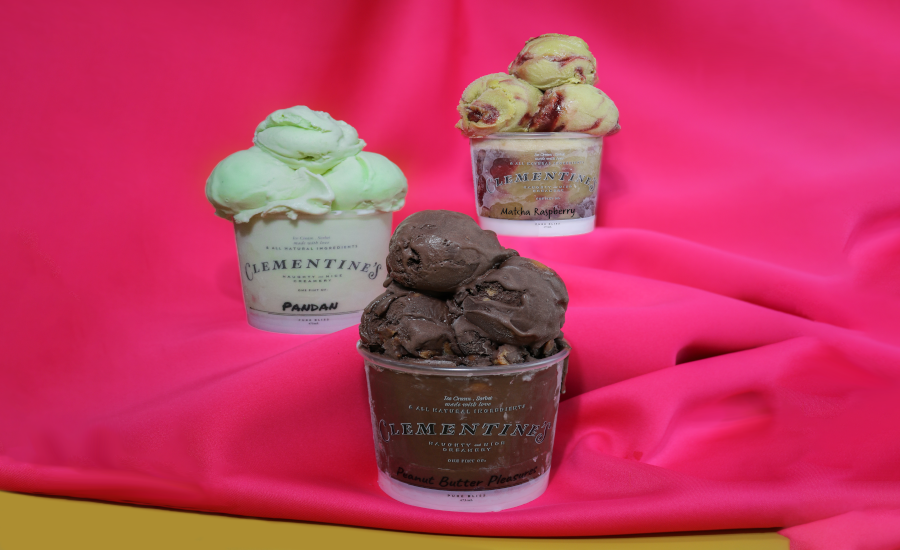This vibrant photograph showcases an artistic setup of three tubs of Clementine’s ice cream, elegantly displayed on a crumpled hot pink satin cloth with a tan-yellow background peeking from the bottom. In the foreground, prominently positioned, is a tub labeled "Peanut Butter Pleasures," featuring several scoops of rich, dark brown chocolate ice cream with potentially creamy peanut butter pieces embedded within. To the left and slightly behind, a second tub contains scoops of a pale green pandan-flavored ice cream, each tub bearing the discernible Clementine’s branding. In the background and towards the right is the third tub, holding scoops of a tantalizing matcha raspberry ice cream, with its yellowish base swirled with vibrant red raspberry streaks. Each tub is overfilled with three scoops, emphasizing the indulgent nature of the ice cream. The carefully arranged scene and contrasting vivid colors of the ice creams and fabric highlight the aesthetics, aiming to attract the viewer's palate and evoke a sense of delicious pleasure.